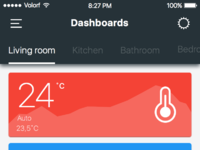A screenshot of a mobile website is depicted, captured from a cell phone. At the very top of the image, a large dark blue rectangle features white text and several icons. On the top left, the word "Volart" is displayed, presumably the name of the cell phone company. Centrally positioned is the current time, "8:27 PM," and on the far right, the battery status reads "100%". Below this, centrally placed, is the word "Dashboards," flanked by a gear icon on the right and a menu button composed of three short lines on the left. At the bottom of the dark blue rectangle, a white underline highlights the "Living Room" tab, with adjacent tabs labeled "Kitchen," "Bathroom," and "Bedroom" in light gray text. 

Directly beneath this section is a large red rectangle positioned prominently within the screenshot. The red rectangle contains white lettering and graphics, displaying "24°C" on the left. Smaller text beneath reads "Auto 23.5°C." To the right of this text, a white thermometer icon is evident. Finally, a long horizontal blue line is situated below the thermometer icon.